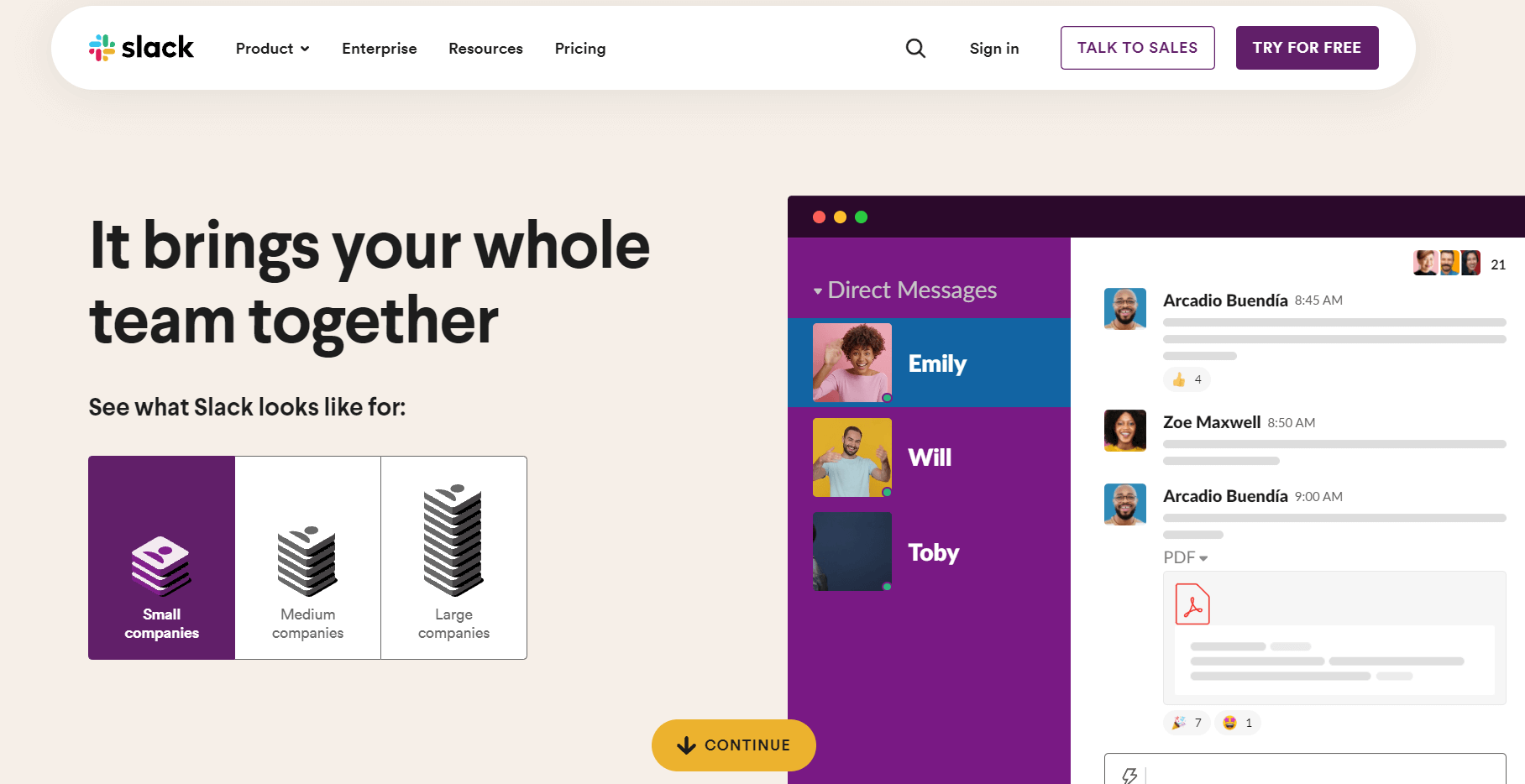The image showcases the homepage of Slack, a team collaboration tool. At the top of the webpage or app, there's a white oval-shaped banner featuring the Slack logo in blue, green, red, and yellow, followed by the word "Slack." The banner also includes a dropdown menu for "Product," and additional options such as "Enterprise," "Resources," "Pricing," a search button, "Sign in," "Talk to Sales," and "Try for Free."

Below the banner, a headline states, "It brings your whole team together," inviting viewers to "See what Slack looks like for." This section is illustrated with images resembling drink coasters, angled to give a dynamic perspective. These coasters represent different company sizes: small, medium, and large, each with a little person icon. The small company area is highlighted in purple, and the coasters increase in size, reflecting the scale of the companies.

To the right, there's an overlay window section featuring direct messages. Here, a purple area displays messages from three individuals: Emily, Will, and Toby. Emily's profile picture shows her with short, curly brown hair, smiling with her left hand raised. She is depicted wearing a three-quarter length, boat-neck style pink T-shirt and has a green availability indicator next to her selfie, which also has a pink background.

Below her, Will's profile shows him against a yellow background, giving a thumbs-up with both hands. He sports a white T-shirt, a beard, and short brown hair, and also has a green availability indicator. Toby, whose image is blank, is listed below them.

Adjacent to these messages, there are additional profile images of people such as Arcadio Buendia and Zoe Maxwell, indicating their availability and participation in the conversation. Arcadio appears twice in this section, each time with an image next to his shared messages.